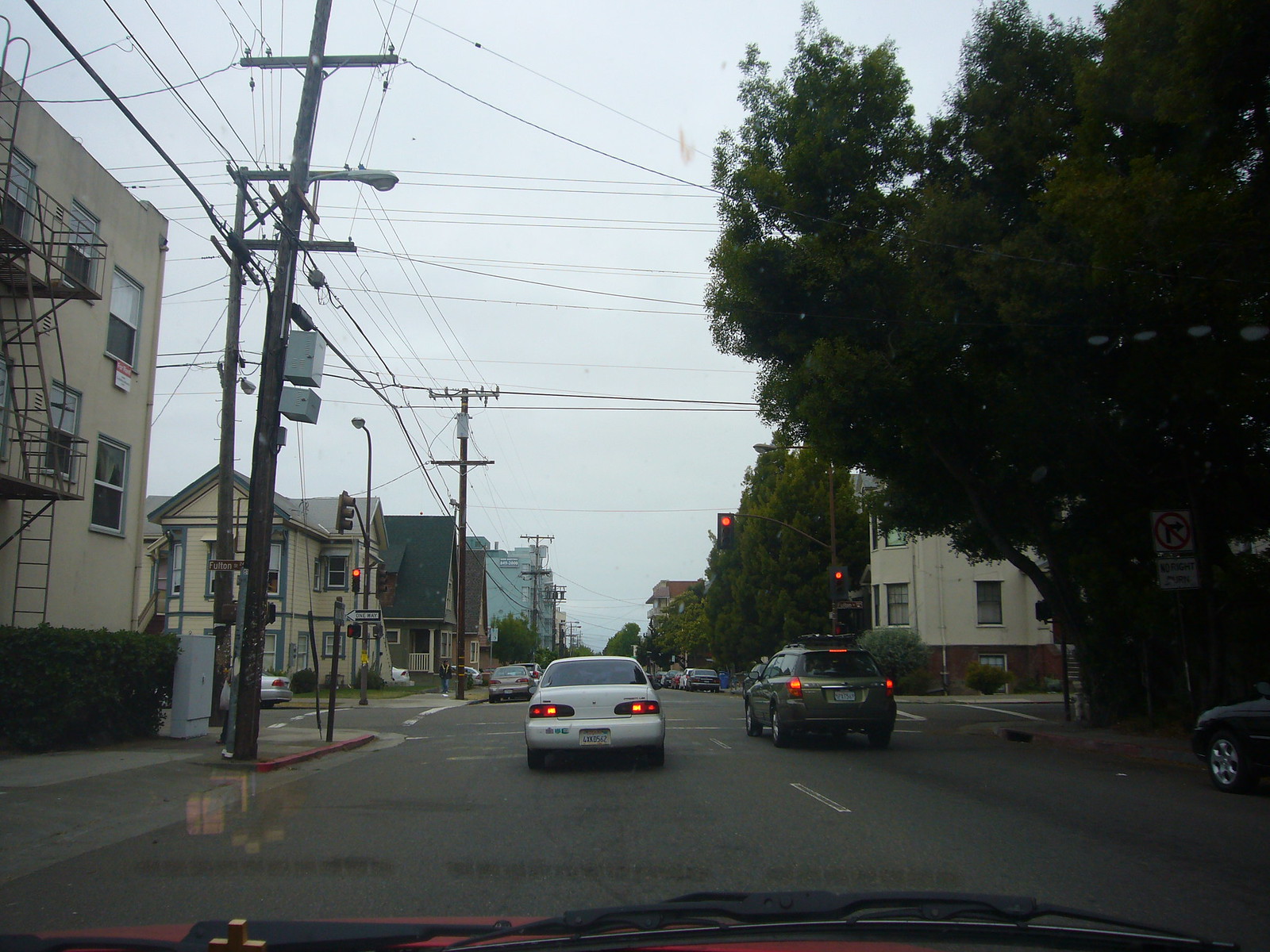A picturesque urban scene captured from inside a car, showcasing a typical neighborhood street. The bottom portion of the image includes a glimpse of the vehicle's dashboard or hood, shaded black. The road ahead is paved with black asphalt, segmented by white lane dividers. In the left lane, a small white car with illuminated taillights waits, its make and model indiscernible. To the right, a gray SUV also displays lit taillights, indicating a halt.

Parked vehicles line both sides of the street, the nearest one on the right partially visible with only its front end in view. A large tree stands prominently, flanking a row of diverse houses. The residences exhibit a mix of construction materials; some are brick, while others feature siding. The houses stretch seemingly endlessly into the distance.

Overhead, a network of telephone wires and poles adds to the urban charm. Further down the street, a traffic light transitions between yellow and red, causing the vehicles to pause. The sky above is overcast, casting a gray hue over the entire scene, adding a tranquil, almost contemplative atmosphere to the snapshot.